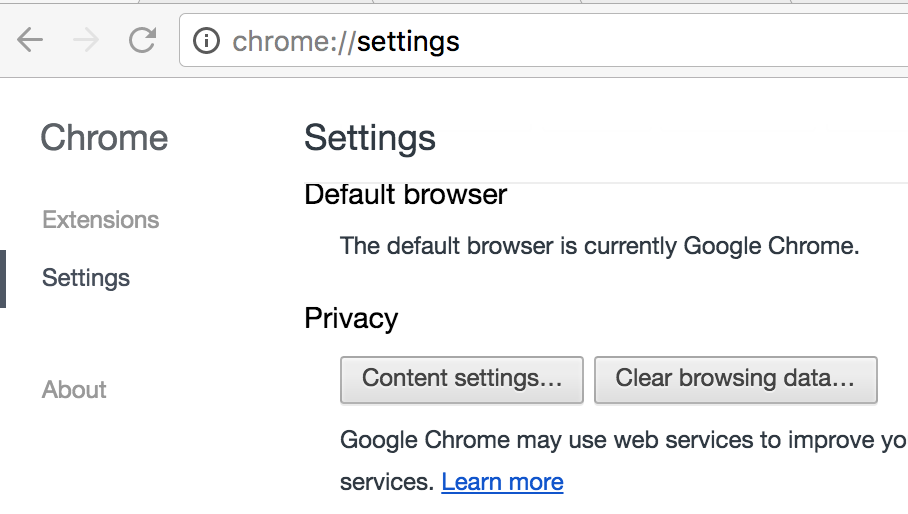This image presents a detailed view of the Google Chrome settings page, focused on a tightly cropped area that highlights specific interface elements. The visible section primarily features the top URL bar, which is a very light gray tone. Notably, the back button is highlighted while the forward button is grayed out. Adjacent to these is the reload button, followed by the URL field displaying "chrome://settings".

Beneath the URL bar, the interface reveals a white background with the settings menu. In this menu, three options are listed: Extensions, Settings, and About, with "Settings" currently selected, evidenced by a prominent black bar to its left. This selection aligns with the main header that reads "Settings" in bold text. Below this heading, the first visible section is labeled "Default browser,” stating that Google Chrome is the current default browser.

Further down, the "Privacy" section is displayed, featuring two gray buttons labeled "Content settings" and "Clear browsing data." The text just below this section reads, "Google Chrome may use web services to improve yo..."—indicating that the phrase is cut off, presumably it originally said "your services." A blue hyperlink beside this text says "Learn more."

The overall design and text imply that this image was captured from a high-resolution screen, likely from a PC, though a tablet cannot be ruled out. The clean, well-aliased text enhances the clarity of the displayed options and settings, despite the cropped nature of the screenshot.